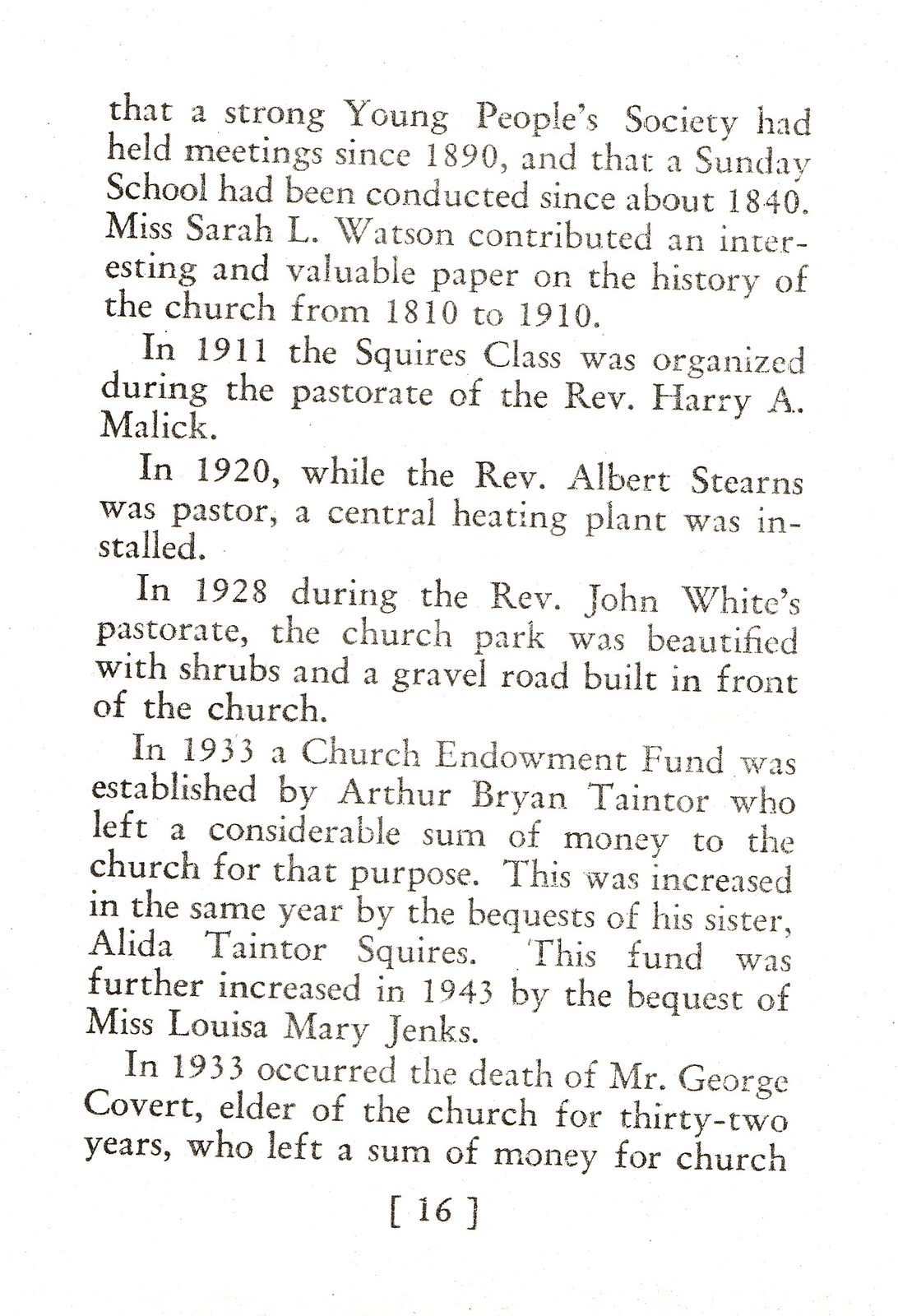This image is a vertically aligned rectangular scanned copy of a book page, featuring five paragraphs of text in black against a white background, with justified alignment. The text highlights several key historical dates and events of a church. It states that a strong young people's society had held meetings since 1890 and that a Sunday school had been conducted since about 1840. Ms. Sarah L. Watson contributed an interesting and valuable paper on the history of the church from 1810 to 1910. In 1911, the Squires class was organized during the pastorate of the Rev. Harry A. Malick. In 1920, while the Rev. Albert Stearns was pastor, a central heating plant was installed. In 1928, under the guidance of the Rev. John White, the church park was beautified with shrubs and a gravel road built in front of the church. By 1933, a church endowment fund was established by Arthur Brian Taintor, with additional contributions from his sister, Alida Taintor Squires, and further increased in 1943 by Miss Louisa Mary Jenks. It also chronicles the death of Mr. George Covert, an elder of the church for 32 years, who left a sum of money for the church. The page is marked with the number 16 at the bottom middle.